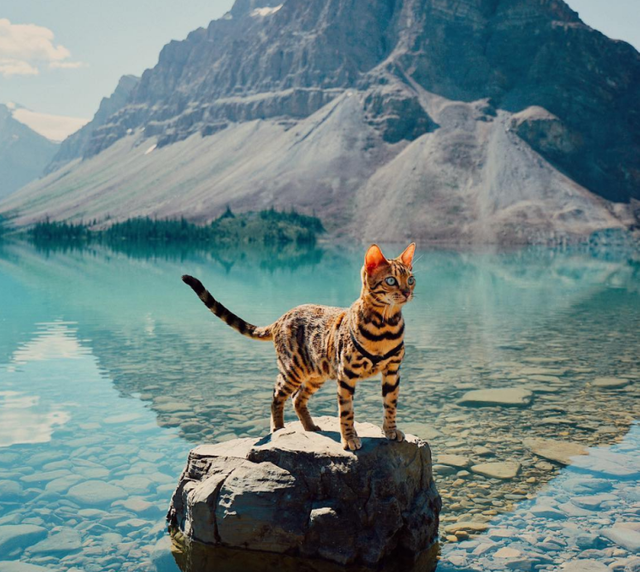In this captivating photograph, an orange tabby cat with distinctive black stripes and striking blue eyes stands gracefully on a large rock in the middle of a pristine, clear lake. The waters, light blue and as transparent as glass, reveal a bed of variously sized rocks beneath its calm, reflective surface. Framing this serene scene, a towering stone mountain stretches from one side of the image to the other, rising majestically until it vanishes at the top center. The rugged mountain is dotted with evergreen trees at its base, giving way to a cascade of rocks that tumble down into the tranquil lake. The cat, slender and long with a particularly alert posture, peers off into the distance, adding a touch of life to this mesmerizing natural landscape.